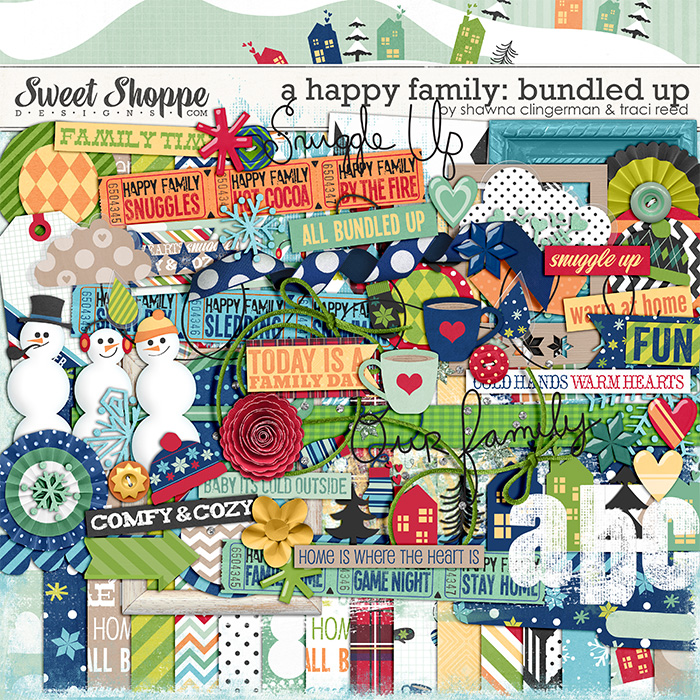This vibrant and festive animated collage, appearing like an advertisement, features a myriad of Christmas-themed elements. At the top, a white banner in cursive reads "Sweet Shop Designs.com," and alongside it, the text "A Happy Family Bundled Up by Shauna Klingerman and Tracy Reed" is prominently displayed. Beneath the banner, the collage brims with a delightful assortment of animated objects and phrases, creating a busy and lively scene.

At the heart of the collage are three distinct snowmen: one with a black hat and pipe, another in the middle with earmuffs and a carrot nose, and a third wearing a cap. Surrounding these charming characters are various holiday-themed items such as tickets with inscriptions like "Game Night," "Stay Home," and "Family Time," alongside coffee mugs adorned with hearts.

The background features Christmas patterns reminiscent of wrapping paper, snowflakes, hearts, and picturesque Christmas sceneries. Scattered throughout the collage are heartwarming phrases like "Comfy and Cozy," "Home is Where the Heart Is," "Snuggle Up," "Warm at Home," "Cold Hands, Warm Hearts," "Family Time," "All Bundled Up," "Baby, It's Cold Outside," and "Today is Family Day." These elements are intricately layered, creating a richly textured and visually engaging holiday scene.